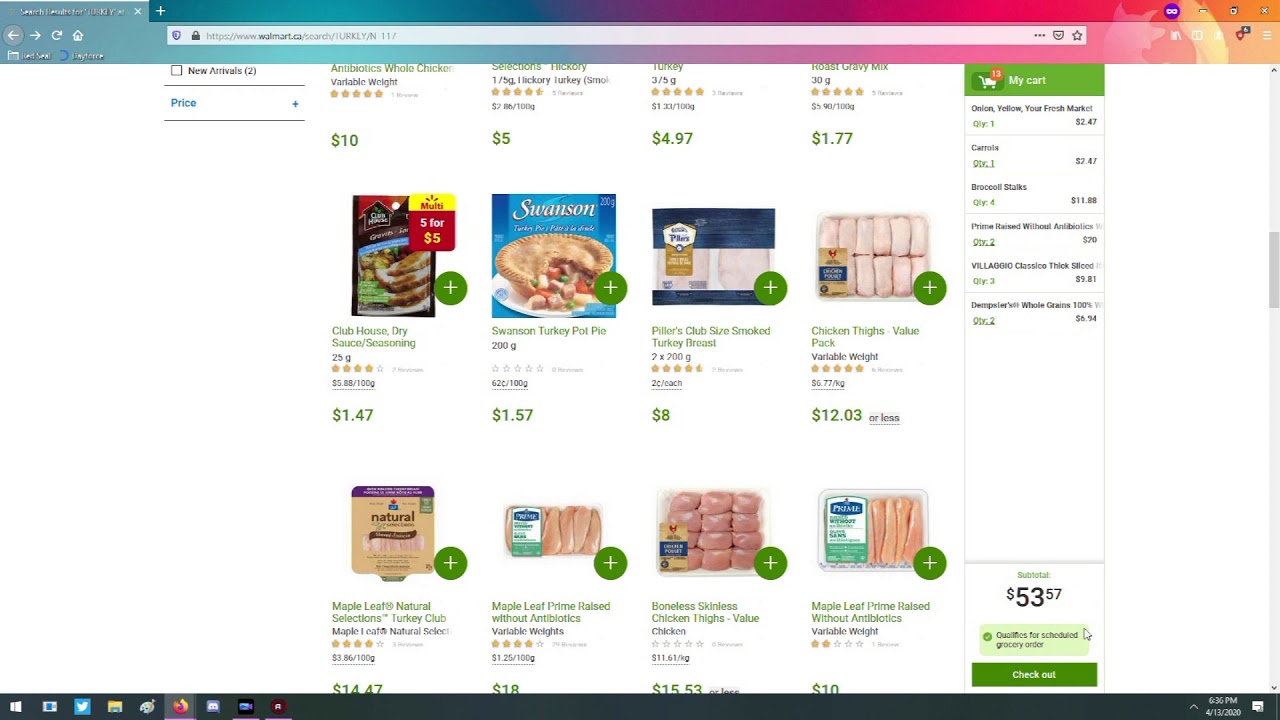In this image, we see a screenshot of a computer screen displaying an online grocery shopping interface. The central area features high-resolution images and detailed descriptions of various food products. Prominently displayed is a rectangular section highlighting a promotion for Clubhouse Dry Sauce Seasoning, available at a special rate of 5 packs for $5 or individually for $1.47 each.

Below this featured offer, there's a Swanson Turkey Pot Pie priced at $1.57, a package of smoked turkey breasts for $8, and a value pack of chicken thighs priced at $12.03. The subsequent row showcases an assortment of items including Natural Selections Turkey Club, antibiotic-free chicken varieties, additional chicken thighs, and prime raised chicken without antibiotics.

In the top right corner of the screen, the viewer's shopping cart is visible. The cart contains various items such as an onion, carrots, broccoli stalks, chicken, and another set of chicken. The precise contents of one additional item in the cart are indiscernible. The bottom right corner of the screen indicates the current total expenditure, which amounts to $53.57.